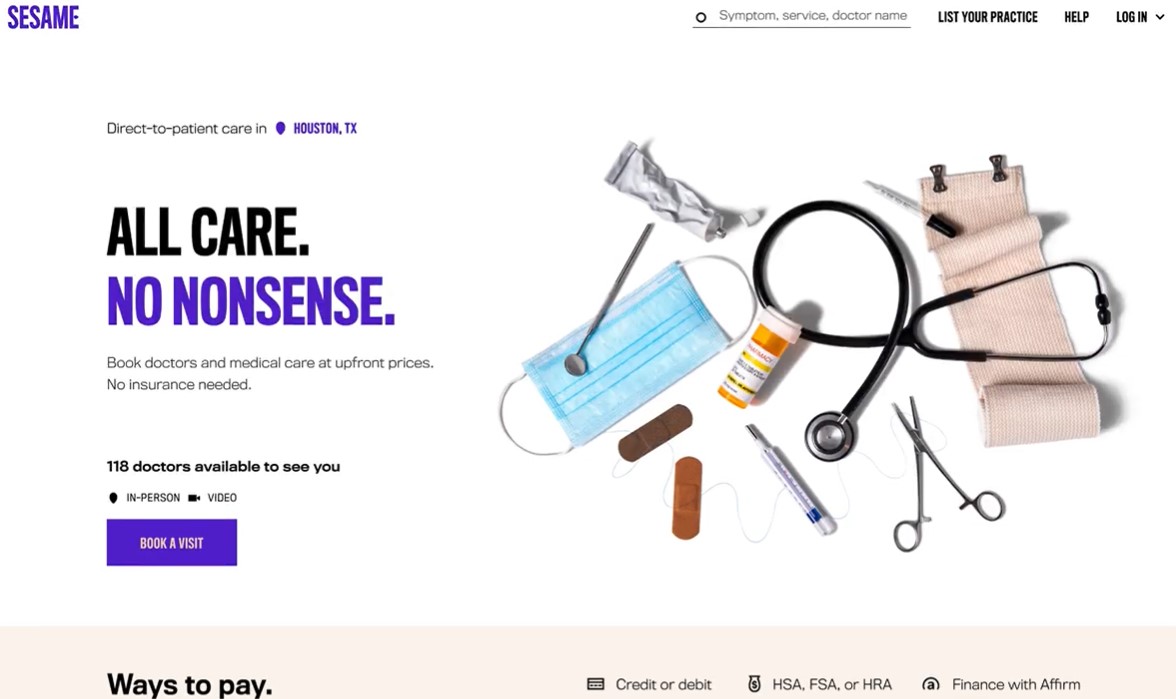This image is a screen capture from the website Sesame. In the top left corner, "Sesame" is prominently displayed in purple font. On the top right, there is a search bar with placeholder text reading "Symptom, Services, Doctor Name." Adjacent to it, bolded in black font, are the options "List Your Practice," "Help," and "Log In," the latter featuring a drop-down arrow.

The main section of the screen showcases a clean, white background. The upper left section headlines "Direct to Patient Care in Houston, Texas." Below, key points are highlighted: “All Care, No Nonsense,” “Book Doctors,” “Medical Care at Upfront Prices,” “No Insurance Needed," and “118 Doctors Available to See You, In-Person or Video.” A prominent purple button labeled "Book a Visit" is also present.

To the right, there is an array of medical equipment, including a stethoscope, pliers, scalpel, pill bottle, band-aids, mask, small mirror, tourniquet, eyedropper, and a tube of medication.

At the very bottom, a tan-colored banner outlines various payment methods: “Ways to Pay: Credit or Debit, HSA, FSA, or HRA, and Finance with Affirm.”